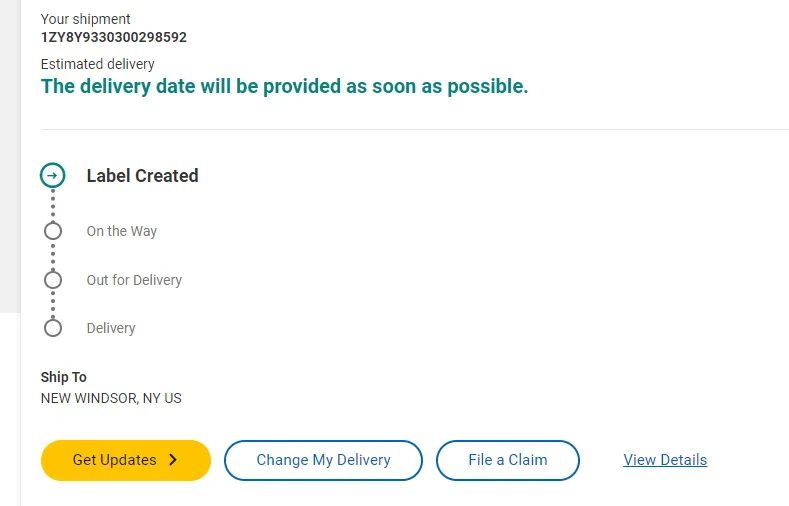Here is a cleaned-up and detailed caption for the image:

---

The image depicts a shipment status update. At the top, the heading "Your Shipment" is prominently displayed, followed by the tracking number: 1ZY8Y9330300298592. Below that, it states "Estimated Delivery" with a note that the delivery date will be provided as soon as possible. On the left side of the image, there's a vertical sequence of four connected circles, each linked by dotted lines. 

1. The top circle, outlined in blue with a rightward-pointing blue arrow, is labeled "Label Created."
2. The second circle bears the label "On the Way."
3. The third circle reads "Out for Delivery."
4. The fourth and final circle is marked "Delivered."

Beneath this section, there is text stating the shipment destination: "Ship to: New Windsor, New York, US."

At the bottom of the image, there are three prominent oval buttons:
  - The first button on the left is yellow and labeled "Get Updates" with a rightward-pointing arrow.
  - The middle button is white with a blue outline and reads "Change My Delivery."
  - The rightmost button is also white but says "File a Claim."

Additionally, in the bottom right corner, there is an underlined link that states "View Details."

---

This detailed caption provides a thorough description of the shipping status image.